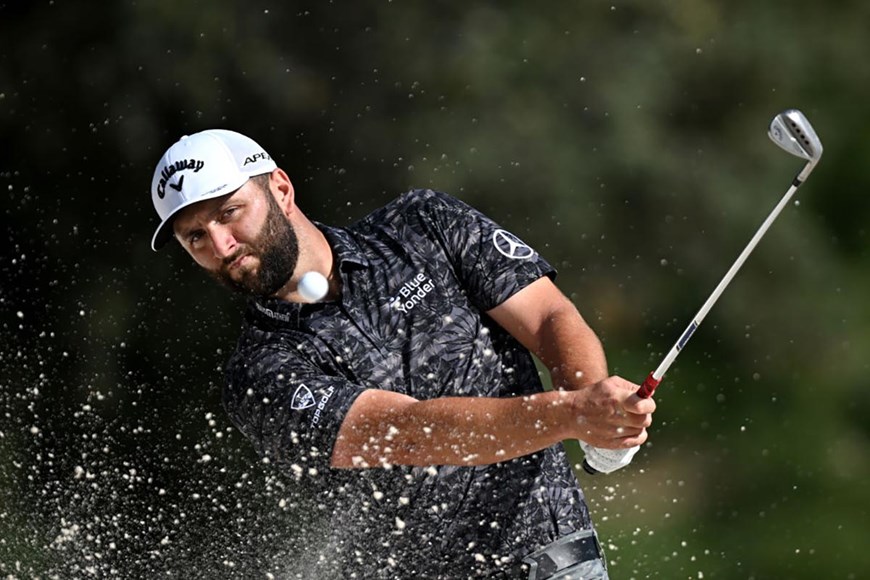This detailed photograph captures a golfer mid-shot in a sand trap at what appears to be a golf course, indicated by the blurred greenery in the background. The golfer, a fair-skinned man with a dark brown beard, is wearing a white Callaway cap featuring a small black "V" logo beneath the brand name. His face is scrunched in concentration as he watches the golf ball soar through the air. He is dressed in a dark gray, striped polo shirt adorned with a Mercedes logo on the left shoulder and a "Blue Yonder" logo on the left chest. Additionally, there is another logo visible on his right shoulder. The golfer wears a white glove on his left hand, gripping a white golf club with a red handle and metallic shaft. At the bottom left of the image, a spray of white sand or foam is shooting upwards, evidence of the powerful swing he has just completed. The golf ball, clearly in mid-flight, is level with the man's neck. The overall composition and blurred background emphasize the intense focus and dynamic action of the shot.